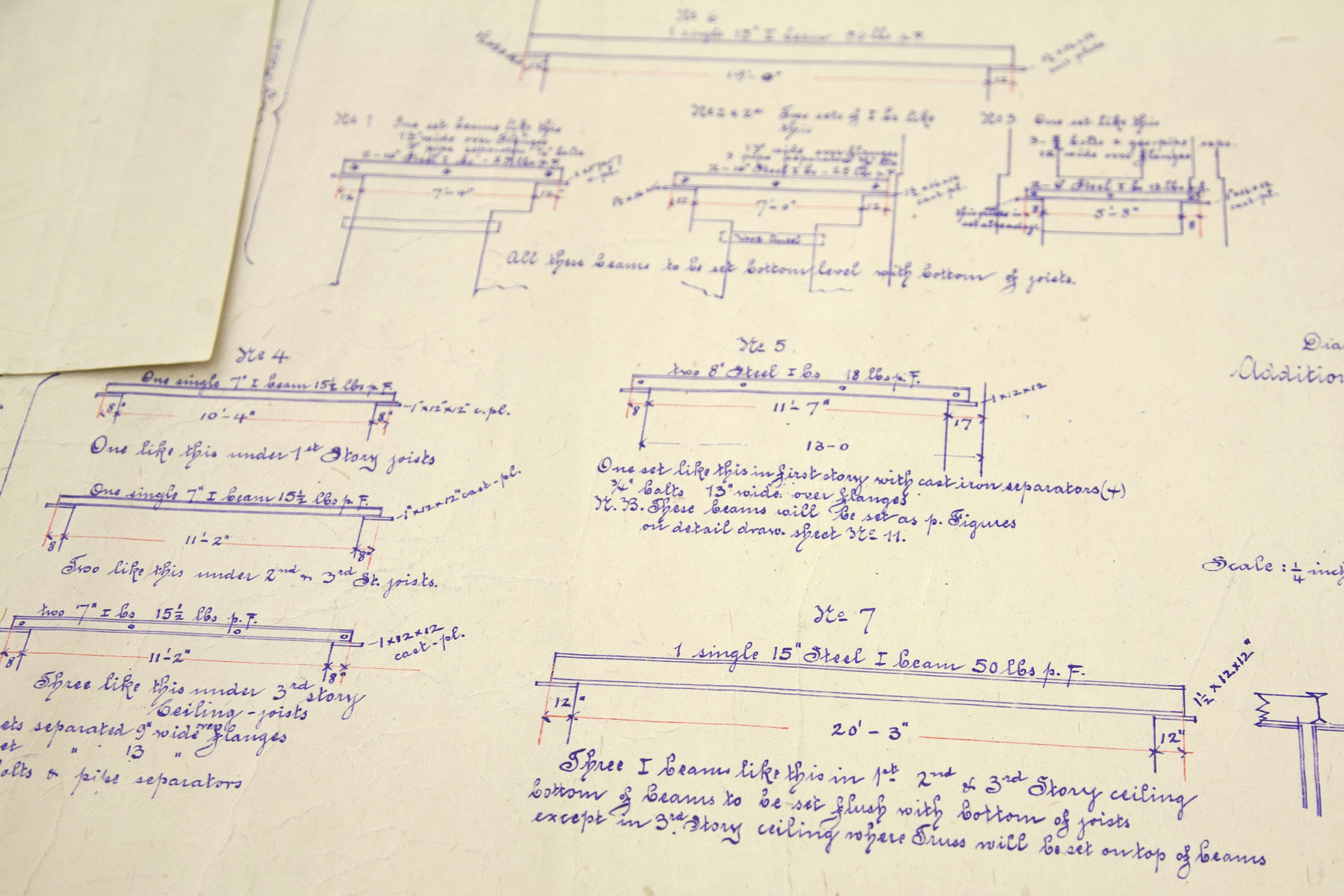The image features a complex set of pen sketches on aged cream-colored paper, showcasing detailed architectural and engineering drawings. The ink used is primarily dark blue or purple, with red lines accentuating measurements. The drawings are a meticulous representation of boards and I-beams, each meticulously annotated with notes and numerical data indicating overall and specific measurements. A prominent long I-beam is positioned at the top, with three others beneath it, all laid out with measurements detailing their lengths, widths, and placements. Despite the illegibility of much of the cursive script below, it is evident that several explanatory phrases and repeated words aim to describe the application and specifications of the beams. One notable annotation reads "single 15-inch steel I-beam, 15 pounds," detailing a beam with a total length of 20 feet 3 inches. Additionally, there are approximately seven individual diagrams depicting various I-beams and truss systems, each varying in length and accompanied by specific notations. The overall depiction suggests these drawings are intended to measure and analyze the load-bearing capacities of these I-beams in construction projects, likely for multi-story buildings.